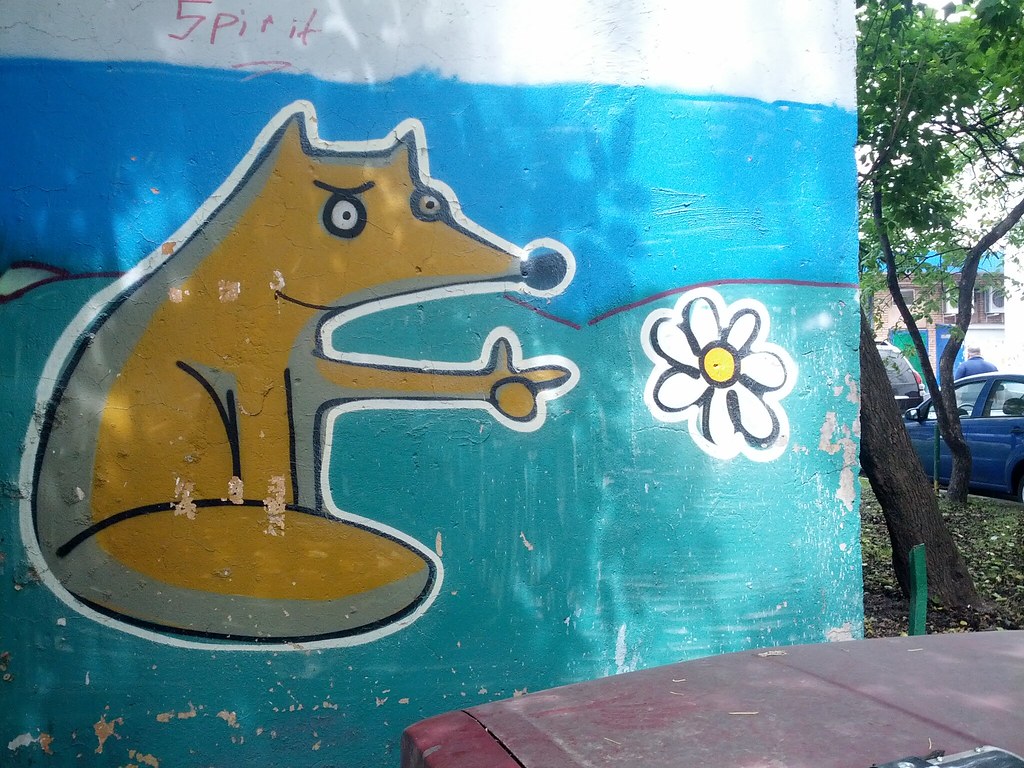The image showcases a vibrant mural on the side of a building, depicting a stylized, cartoonish yellow-brown fox with a friendly smile and expressive black eyes, characterized by large black pupils and white sclera. The fox, outlined in black and further highlighted by a white contour, sits on the left side of the mural on a teal-colored grassy ground against a blue sky background. The fox's left paw is extended, with its pointer finger and thumb raised, gesturing towards a large, daisy-like white flower with seven petals and a bright yellow center, outlined similarly in black and white.

Above the fox's head, the word "spirit" is painted. The mural's background features a light bluish-green area resembling a hill separated from the blue sky by a black dividing line. To the far left, curved lines suggest additional hills. The outdoor scene captured in the photograph includes a bit of the surrounding environment: a tree with green leaves, part of a blue car, the hood of a red car, and buildings in the background, along with a person walking on the sidewalk.